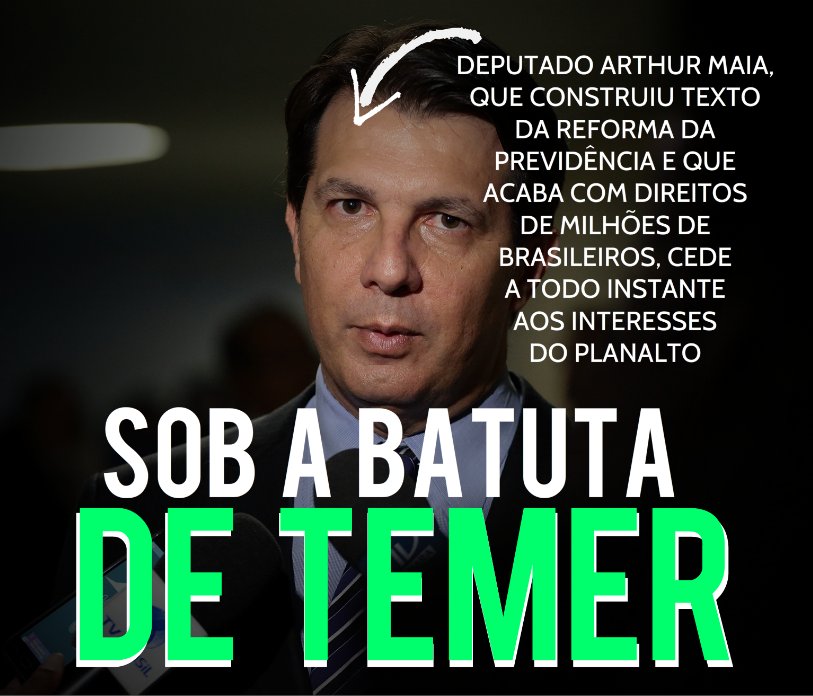In the center of this square image, there is a headshot of a middle-aged white male with dark hair and eyes, likely in his mid to late 50s. He is wearing a dark suit, a light blue shirt, and a striped tie. The background is very dark, almost black, with indistinct shadows and lights that suggest people or shapes behind him, and someone is holding a microphone close to his face, indicating he is being interviewed. 

An arrow points towards his forehead, leading to a block of approximately ten lines of text to the right of his head in Brazilian Portuguese. The text reads "Deputado Arthur Maia que construiu o texto da reforma da Previdência e que acaba com direitos de milhões de brasileiros e dá todo instante aos interesses do Planalto." Below his chin, in large white letters, is written "Sob a batuta de Temer,” with “de Temer” highlighted in green, outlined in white, giving a three-dimensional effect.